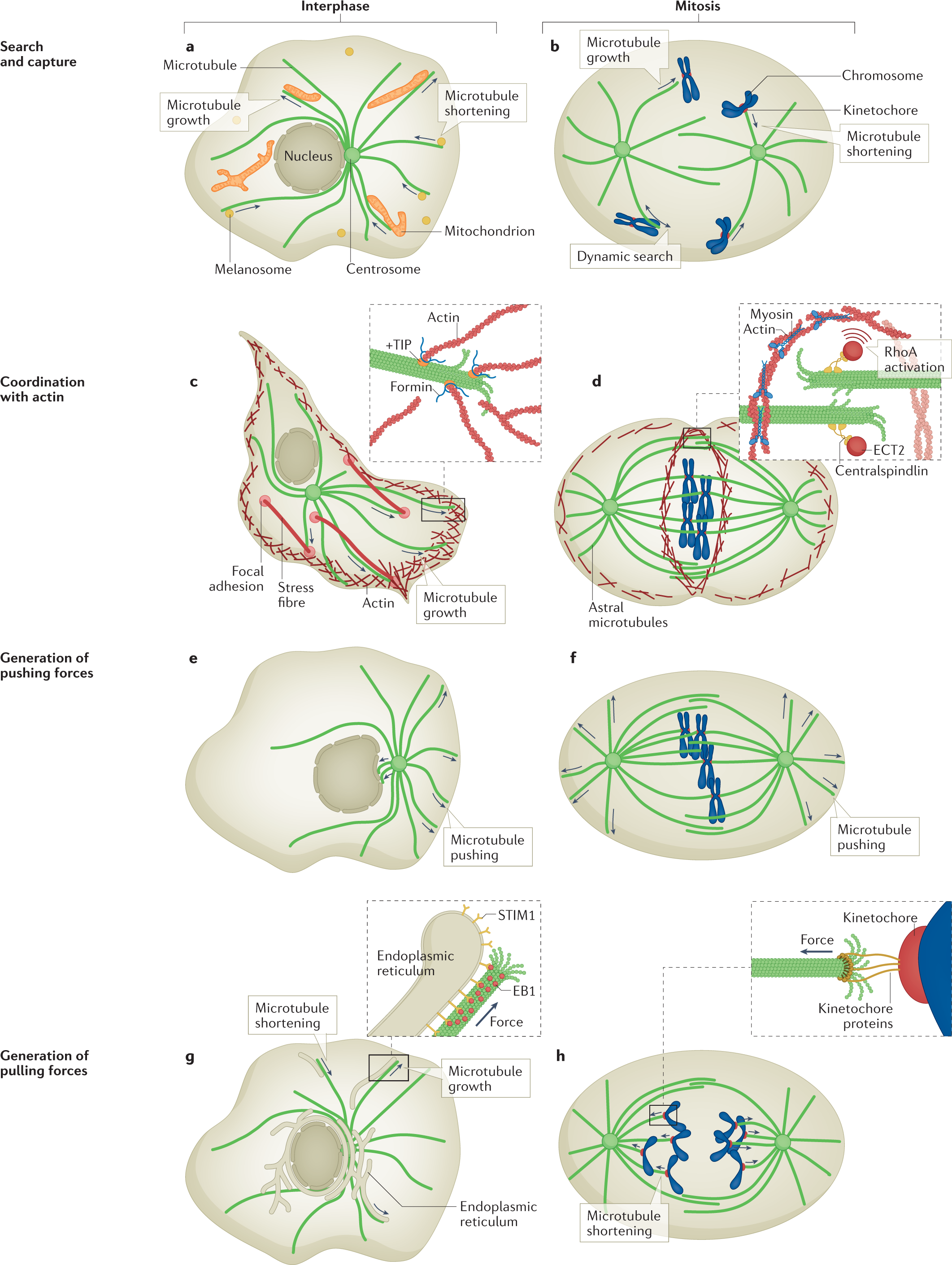This image is a detailed scientific flowchart illustrating the stages and mechanisms involved in cellular division, specifically interphase and mitosis. The flowchart consists of eight diagrams arranged in two columns and four rows, labeled alphabetically from A to H. The diagrams depict processes such as search and capture, coordination with actin, the generation of pushing forces, and the generation of pulling forces, running from top to bottom. Key cellular structures like chromosomes, mitochondria, and microtubules are highlighted in various colors—chromosomes in blue, mitochondria in red, and microtubules in green. The overall color scheme is a mix of beige for the cell structure and nucleus, with accented colors to enhance clarity. The detailed diagrams, accompanied by tiny writing, suggest the image is likely sourced from a biology textbook, aiming to provide an in-depth understanding of cellular mechanics.